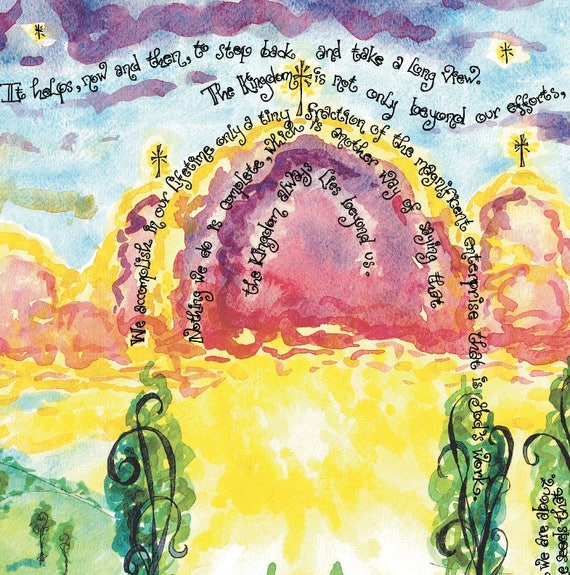The image is a vibrant watercolor with dominant hues of yellow, pink, and purple. It showcases a serene scene with three domes, each crowned with a cross, capturing a spiritual essence. Flowery, flowing black ink forms a thoughtful text that starts horizontally and curves around the central dome, reading, "It helps now and then to step back and take a long view. The kingdom is not only beyond our efforts. We accomplish in our lifetime only a tiny fraction of the magnificent enterprise that is God's work. Nothing we do is complete, which is another way of saying that the kingdom always lies beyond us." The lower part of the painting introduces a pastoral landscape with tall trees and two smaller trees on the bottom left, bathed in a purplish light, possibly reflecting the setting sun. A beam of yellow light touches the ground, emphasizing the ethereal feel of the artwork. Purple clouds scatter across a blue sky, harmonizing with the earthly scene, completing this intricate and hopeful tableau.